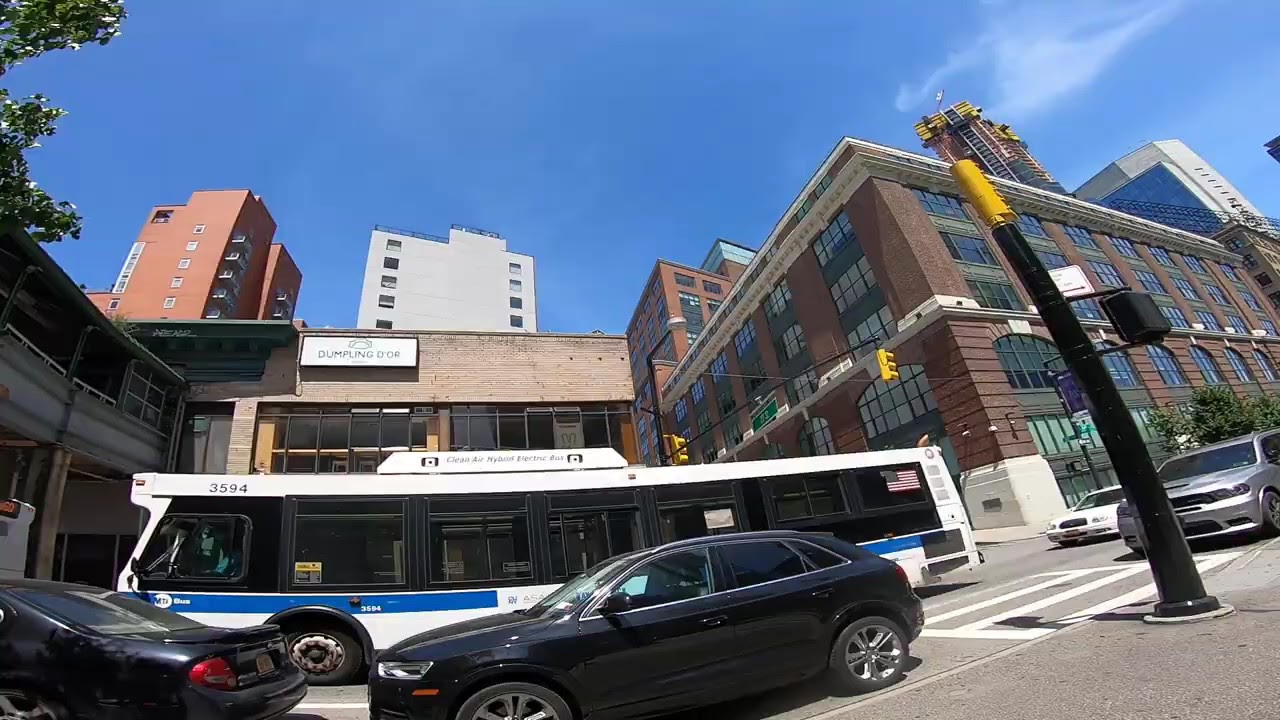This daytime city street scene captures a bustling urban environment under a beautiful blue sky with a few hints of white clouds. Prominently featuring a mid-sized brick building with many windows, likely around six to seven stories tall, the photo also showcases towering apartment complexes in the background, some reaching 20-30 stories. On the busy road, a large white bus with a blue stripe stands out, accompanied by two black cars traveling in the same direction, followed by a sequence of a white car and a silver car. Street signs and traffic lights are visible, along with a crosswalk crossing the road. The vibrant street is dotted with various trees along the sidewalks, adding to the urban greenery. Notably, a brick building with a sign reading "Dumpling D'Or," possibly a restaurant, is present, enhancing the city's cultural texture. Lastly, a black pole with yellow markings adds another touch of urban infrastructure to this picturesque and sunny city moment.